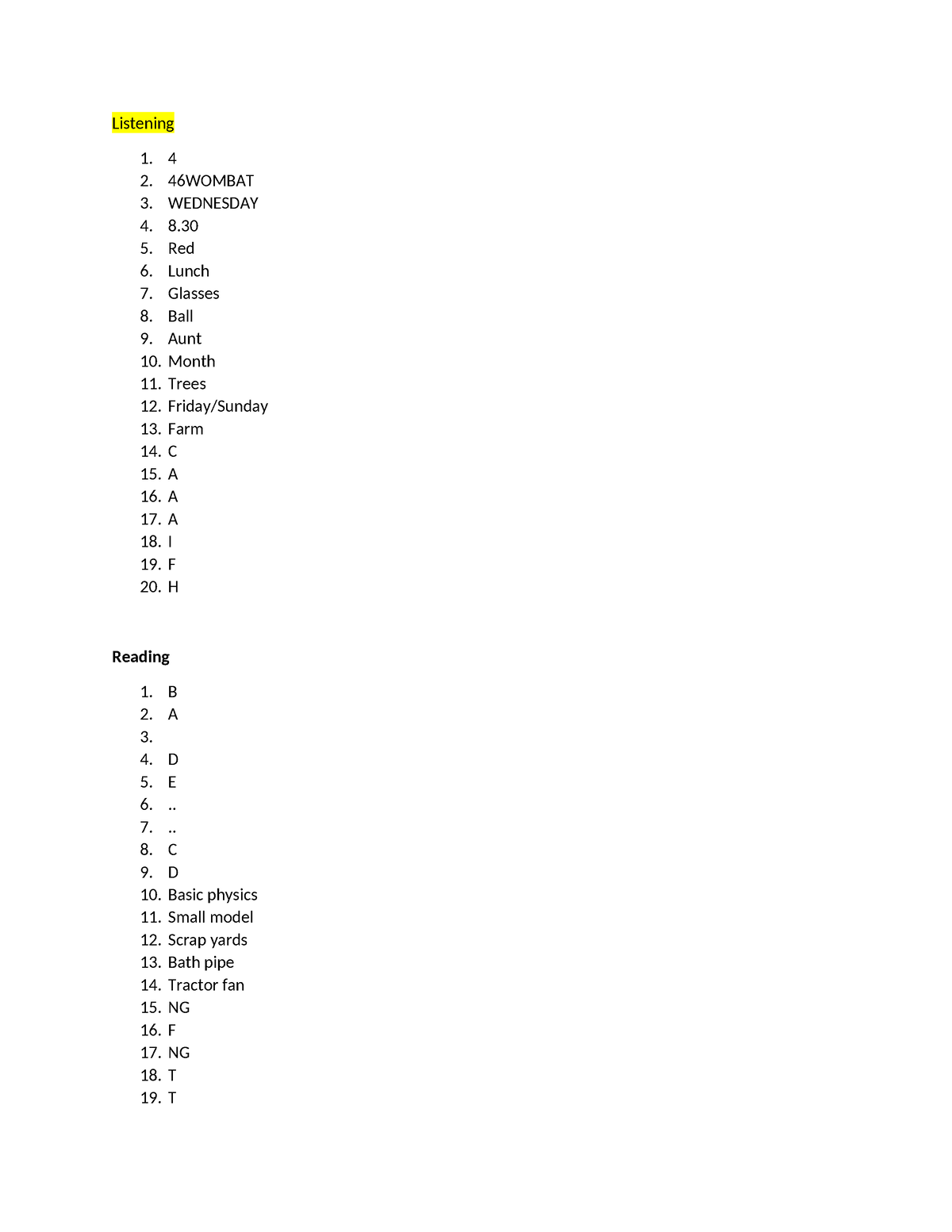This image depicts two vertically listed categories of information against a white background with black text. The first category, titled "Listening" and highlighted in yellow, is numbered from 1 to 20. Each number is accompanied by specific words or phrases: 4, 4-6 Wombat, Wednesday, 8:30, Red, Lunch, Glasses, Ball, Ant, Month, Trees, Friday-Sunday, Farm, Sea, A, A, A, I, F, H.

Directly below this is the second category titled "Reading", listed without any highlight and numbered from 1 to 19. The corresponding entries are: B, A, (Blank), D, E, Dot Dot, Dot Dot, C, D, Basic Physics, Small Model, Scrap Yards, Bath Pipe, Tractor Fan, NG, F, NG, T, T.

This appears to be an organized exercise list that differentiates between "Listening" and "Reading" activities, potentially designed for educational or training purposes.